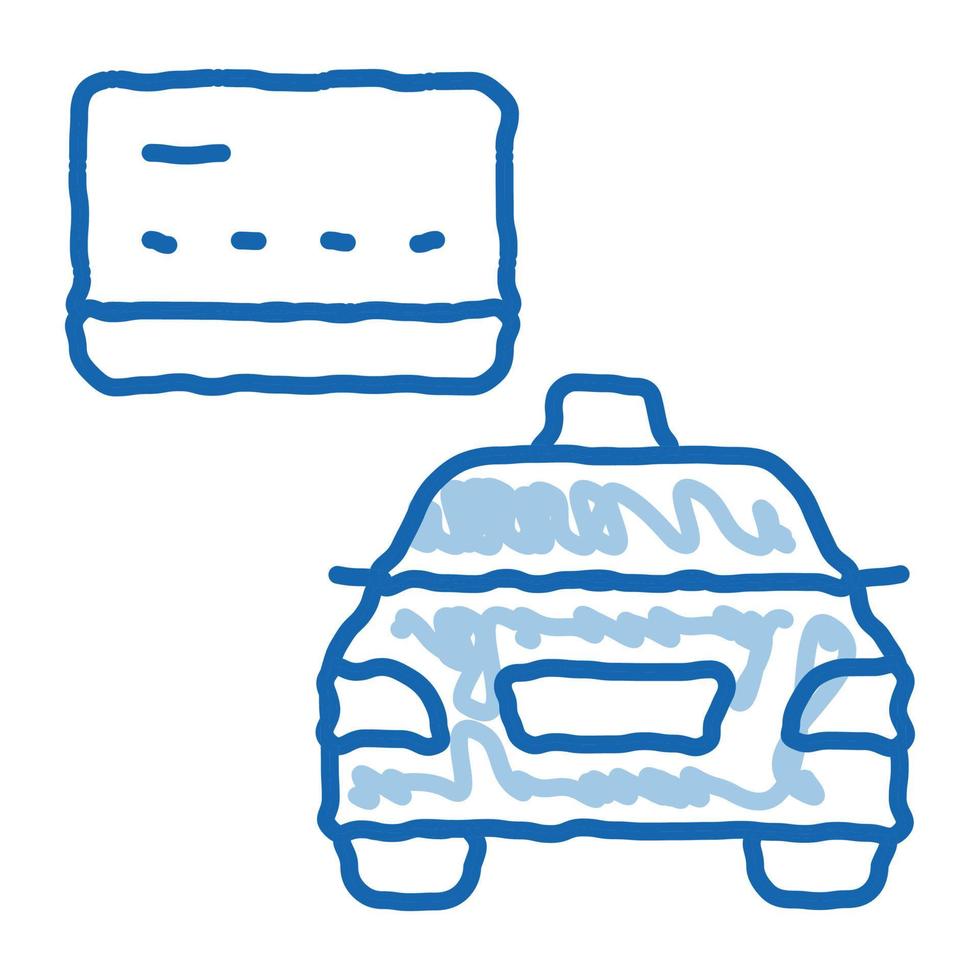The image in question is a cartoonish, hand-drawn depiction featuring two main elements against a white background, both rendered in squiggly dark blue lines with light blue shading. The primary focus is on a vehicle, likely a taxi cab, facing toward the viewer. This is indicated by a small sign on the roof, characteristic of a taxi, along with visible headlights, front grille, windshield, and tires—all defined by the same wavy linework that contributes to the overall whimsical style. The body of the taxi is filled with light blue squiggles adding texture and a hint of color differentiation.

Above and to the left of the taxi, there is a rectangular card-like object that resembles a credit or debit card, complete with a band across its bottom, potentially representing a magnetic stripe. The card also features dashed lines and dots where text or information might typically be found. This abstract portrayal captures the essential shapes and features of both objects, maintaining a cohesive and somewhat crude stylistic execution throughout the image.